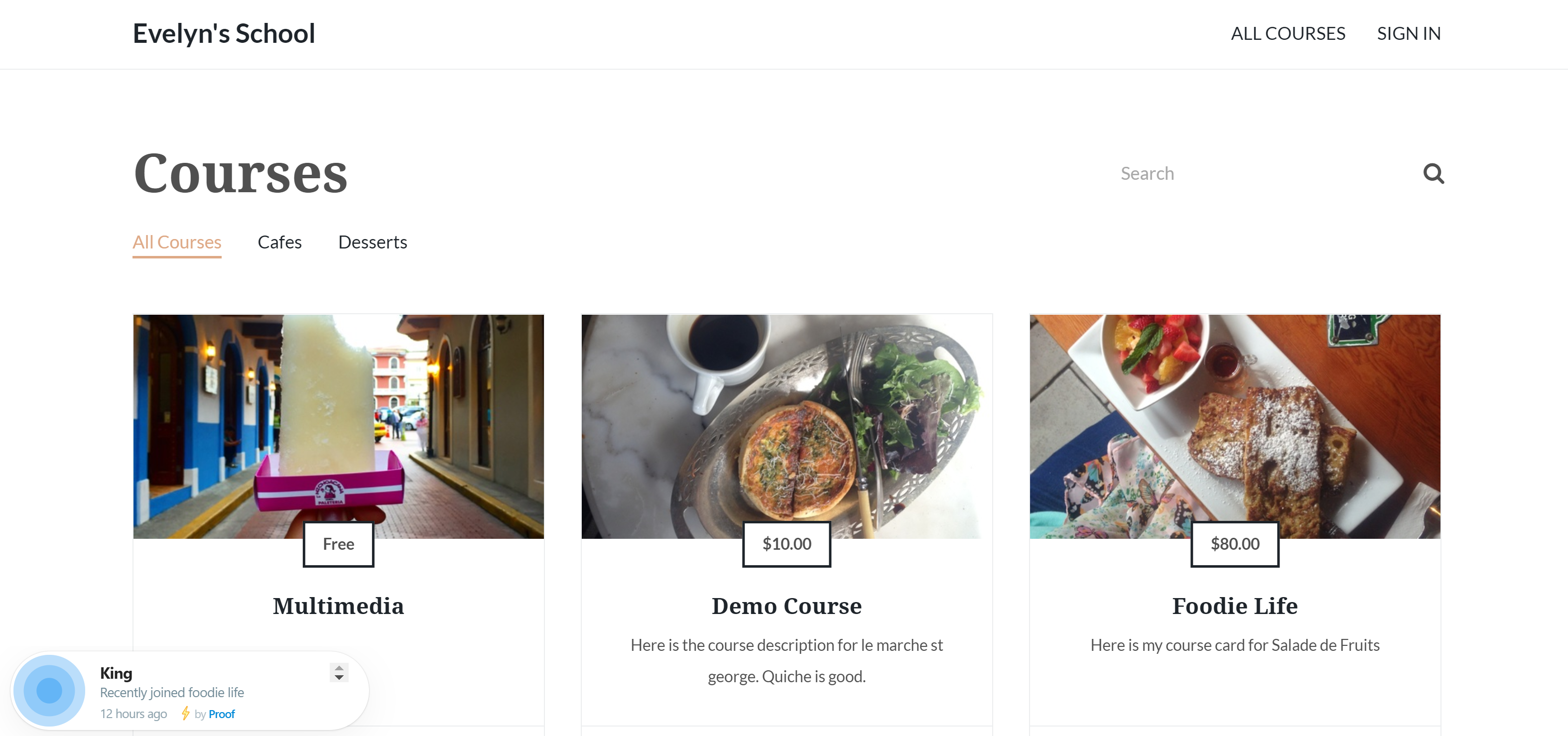Screenshot of Evelyn School Website

The screenshot depicts a section of a website with a clean, white background. At the top left corner, the site is branded with the name "Evelyn School." To the right of this, there are navigational links labeled "All Courses" and "Sign In."

Beneath this, the left section contains a heading titled "Courses" with options such as "All Courses," "Cafes," and "Desserts" listed below it. The "All Courses" option is currently selected and underlined.

Adjacent to the "Courses" heading on the right is a prominent search bar adorned with a search icon.

Further down, there are three rectangular images representing different courses:

1. The first rectangle displays the label "Free" and the title "Multimedia." The image features an alley between two buildings. 

2. The second rectangle shows a plate of food accompanied by a cup of coffee, priced at $10. This entry is titled "Demo Course" with a brief description: "Here's the course description for La Marca at George. Quiche is good."

3. The third rectangle depicts a delectable pastry on a white plate, under the title "Foodie Life," priced at $80. The description reads, "Here is my course card for Salada de Fruits."

Additionally, in the bottom left corner, there is a small blue circle icon accompanied by the word "King," indicating that someone named "King" has recently joined the "Foodie Life" course.